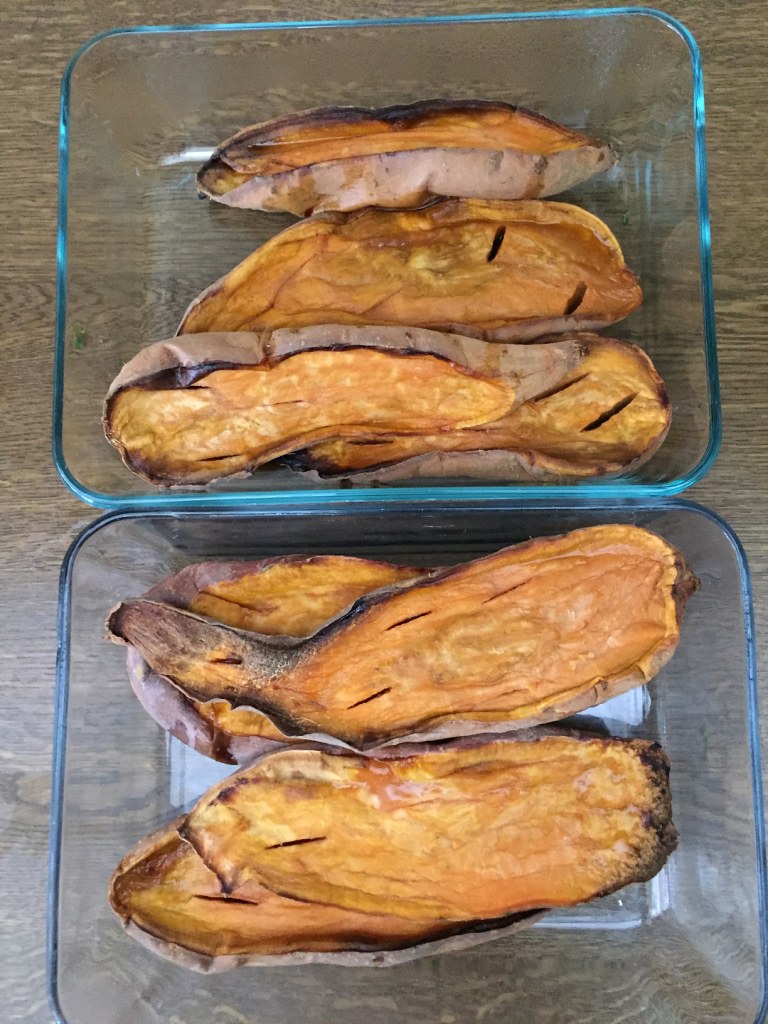The image depicts two translucent, clear glass containers with a slight blue hue around the edges, due to the thickness of the glass. These containers rest on a medium brown wooden countertop or table. Inside each container is a roasted or baked starchy vegetable, resembling a sweet potato or possibly squash. The vegetables are long and oval-shaped with a burnt orange coloring and a browned exterior, possibly from being cooked in the oven. Each vegetable has been cut in half, revealing a yellowish interior with some fine cut marks and edges that are blackened and crisp. The bottom of the containers appears to have a small amount of liquid, likely from the cooking process. The overall impression is of pre-cooked or baked vegetables carefully placed in these glass dishes.